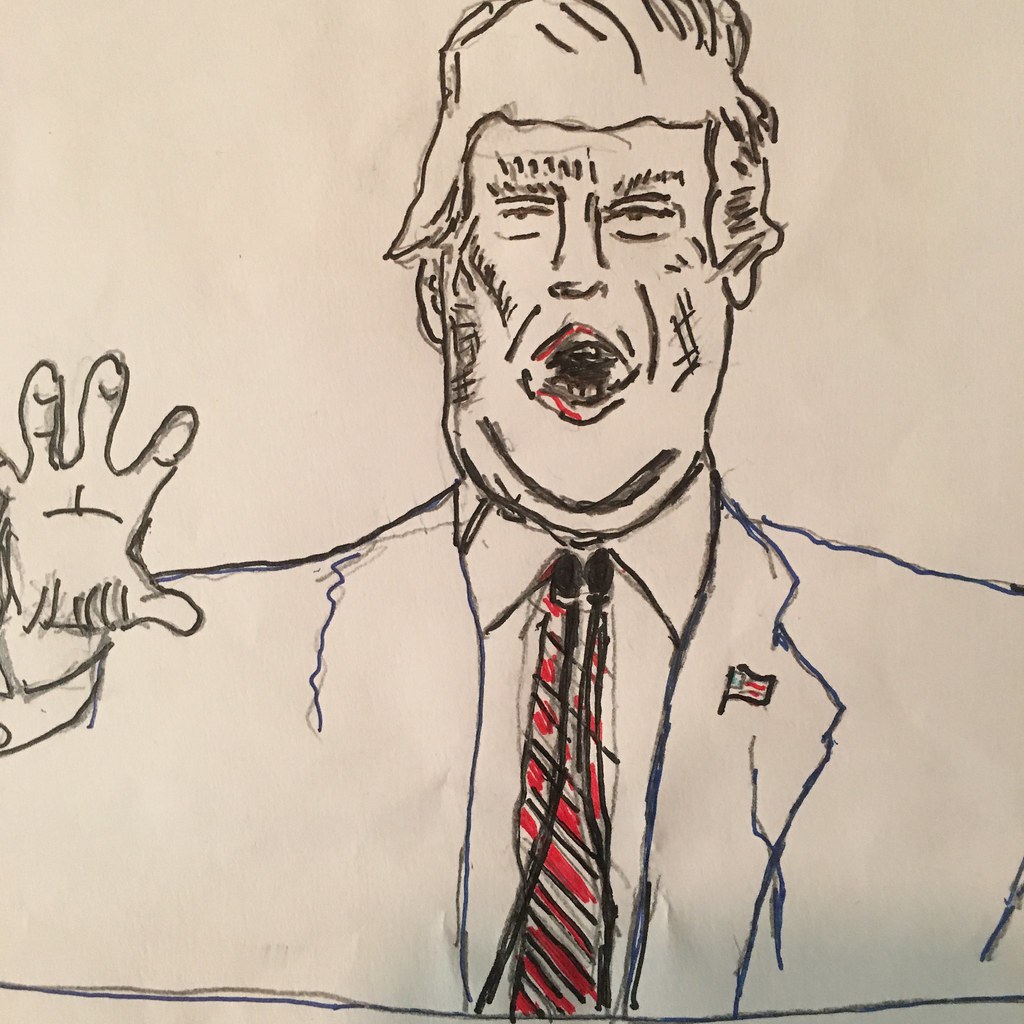This artwork is a stylized, jagged portrait of Donald Trump, seemingly crafted first in pencil and then enhanced with darker ink or markers for emphasis. The figure is depicted in a frontal view, with an outreached palm on the left side of the image, suggesting an inviting or possibly assertive gesture. Trump is attired in a traditional suit jacket that is detailed with blue outlines and is accessorized with a small American flag pin prominently displayed to the left of his red-and-black striped tie. Touches of red accentuate the tie, his lips, and the American flag pin, adding vibrant contrast to the otherwise monochromatic suit. The rough, uneven lines lend a chaotic energy to the composition, capturing a striking and dynamic representation of the former president.